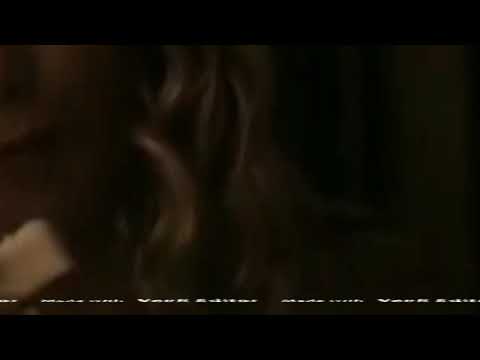This image depicts a murky, out-of-focus scene with various indistinct elements and a predominantly dark palette. At the center and slightly to the left, there appears to be a groove or a break in the continuity of the frame, possibly suggesting depth or segmentation. Protruding from the lower left corner is an ambiguous stick-like object. The image background is lighter on the left side but transitions into darker hues on the right, culminating in an entirely black area where no details are discernible. Highlighted strands of what could be brown hair spread across the middle of the frame, hinting at a human presence. Attached to this is a dark-colored sleeve, extending an arm from the lower left part towards the center. The image is flanked by relatively thick black borders on the top and bottom, and the lower section contains a partially visible and unintelligible caption, fragmentarily suggesting, "made with." The interplay of tan, light brown, white, and black tones adds to the obscurity and ambiguity, making it difficult to determine whether the scene is real or digitally rendered.